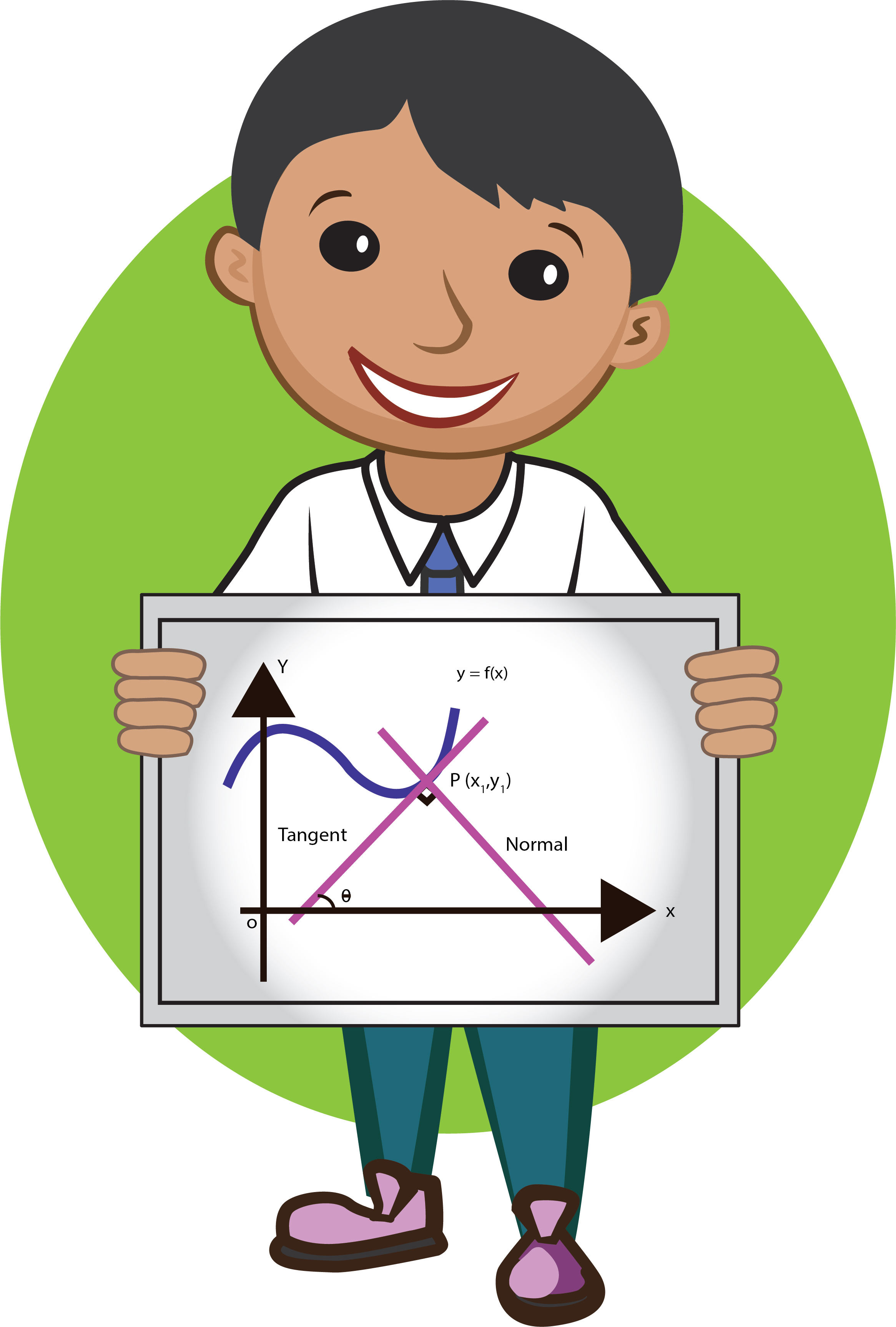This detailed and descriptive cartoon illustration features a man with short, dark hair, possibly of Hispanic descent, smiling warmly. He wears a white dress shirt paired with a blue tie and teal green pants, along with eye-catching purple shoes with a wide base. This character, who might represent a teacher or a student, stands against a lime green background and holds up a poster. The poster prominently features a graph complete with labeled X and Y axes, marked with arrows pointing upward and to the right, respectively. At the intersection of these axes, labeled 'O', the terms ‘tangent’ and ‘normal’ are written on the left and right sides of the graph. The graph also includes a blue squiggly line at the top extending from the Y-axis to the right and two crossing purple lines near the center, forming a shape reminiscent of a pyramid. This vibrant and educational graphic appears targeted towards middle school or high school algebra students, making complex mathematical concepts visually engaging and accessible.